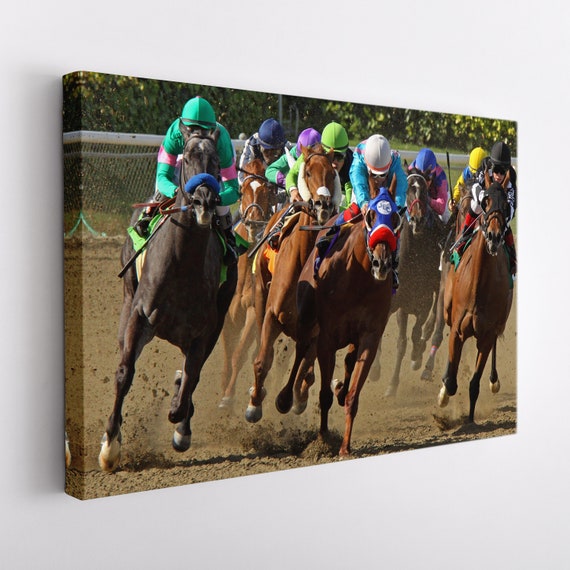The image captures an intense moment in the middle of a horse race on a dirt track, with eight jockeys riding horses in full gallop, coming toward the viewer. The horses vary in color, including shades of brown, dark brown, light brown, and a striking black horse. Dirt is visibly flying up from the track due to the horses' powerful strides. The jockeys are dressed in a variety of colorful outfits and helmets, featuring combinations like medium green, lime green, white, yellow, blue, dark blue, purple, and more. Each jersey either matches or contrasts with its corresponding helmet color, adding a vivid array of hues to the dynamic scene. The photo is a box canvas hanging on the wall, unframed, showcasing the jockeys' intense focus as they lean forward, their helmets and heads down, and the coordinated matching tack on the horses. The visual energy and detail of the jockeys' brightly colored attire and the horses' dynamic motion capture the thrill and fast-paced nature of the race.